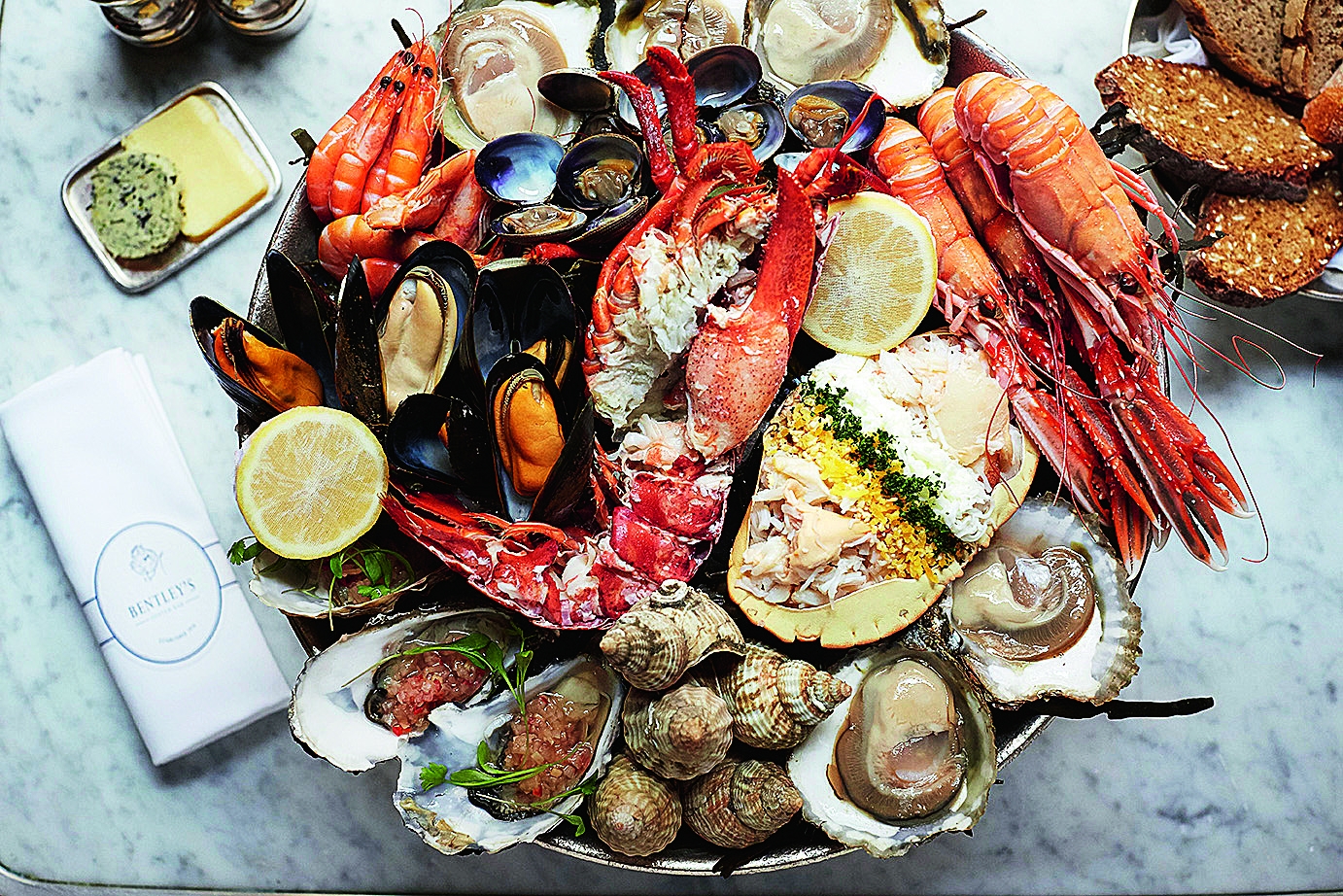An elegant granite table with a bluish-white, marbled surface hosts an abundant spread of seafood. Centered is a grand platter featuring an impressive variety of seafood: oversized prawns, lobsters, crabs, clams, snails, and conches. The extensive selection includes a pair of scallops in their open shells, oysters adorned with a tangy sauce and sprigs of greenery, and lemon halves scattered throughout. Beside this seafood medley is a smaller platter with a selection of cheese. To the right, a bowl contains hearty whole grain bread, and a piece of avocado toast sits nearby with butter. A napkin bearing Bentley's logo is neatly placed on the table, hinting at a luxurious dining experience.